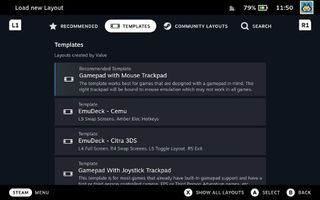In this smartphone screenshot, the [Load New Layout] interface is displayed within a dimly lit application, presumably for a gaming or controller customization app. The user interface features multiple templates for layout customization and a set of navigational tabs at the top of the screen. These tabs, from left to right, are labeled as follows: [Recommended], [Template], [Community Layout], and [Search]. The [Template] tab is prominently highlighted with a white background and black text, indicating it's the current active tab, while the other tabs have a black background with white text.

On the upper corners of the screen, there are controller patterns labeled [L1] on the top left and [R1] on the top right, both in white text, seamlessly blending into the dark background. 

Below the tabs, the interface presents four layout options. The highlighted option is the "Gamepad with Mouse Trackpad," distinguished by a blue line to its left. The description for this layout is marked as blurry. The other layouts listed are titled "Emotech," "Emotech Citra 3DS," and "Gamepad with Joystick Trackpad," though their detailed descriptions remain obscured.

At the bottom of the screen, navigation aids are provided: in the lower left corner, it reads [Steam Menu], while the lower right corner includes several options: [Show All Layout], [Select Back], with [A] for selecting and [B] for going back. 

The layout [created by] information indicates the username "hideth," although this specific detail is somewhat subordinate in the overall interface presentation.